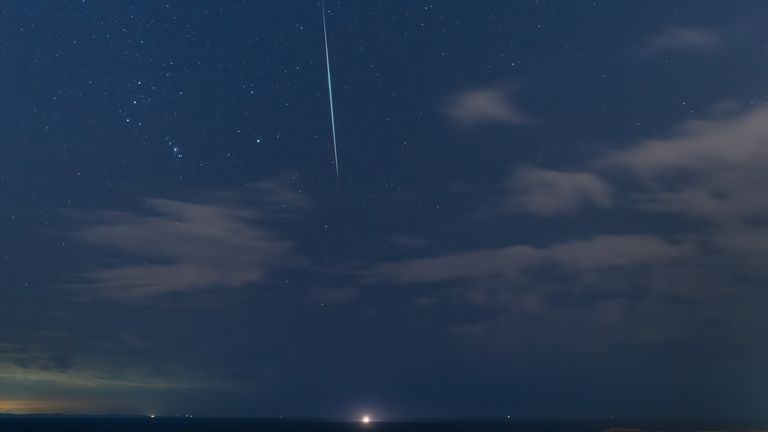This color photograph captures the night sky just after sunset, with the majority of the photo (about 90%) dominated by a mostly clear, dark blue sky sprinkled with stars. A subtle hint of orange from the recently set sun can be seen in the lower left corner. The sky contains some wispy, thin clouds, but remains predominantly clear, allowing a spectacular view of the stars. An intriguing white streak, likely a meteor or possibly an airplane, extends from the top center of the image towards the middle, directing the viewer's eye down to a bright, intense white light at the horizon line, which resembles a spotlight on the land. The ground appears dark, with small specks of light dotting the horizon, giving a sense of depth and scale to the serene night landscape.